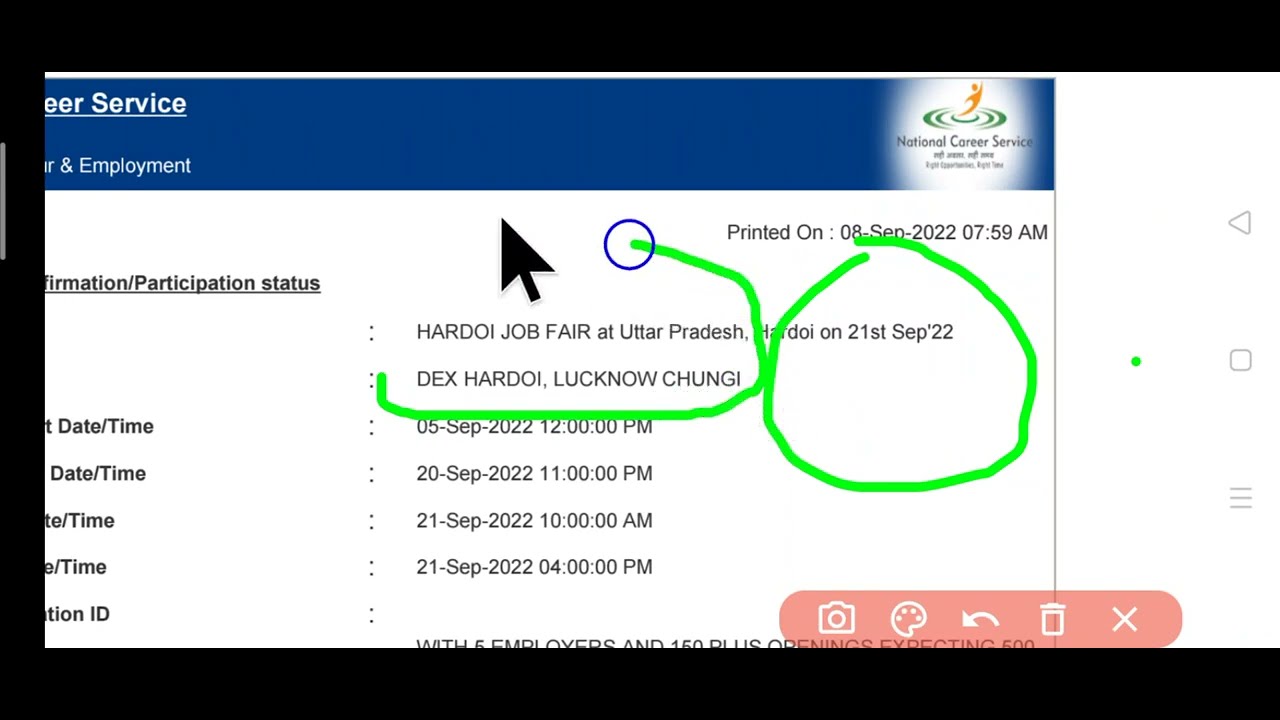This image is a detailed screenshot of a webpage with significant editing and annotations. At the top of the page, there is a blue banner featuring a logo with the text "National Career Service" written beneath it. Dated "08 Sep 2022, 07:59 a.m.," it includes details about a "Hardoi Job Fair" held in Uttar Pradesh on 21st September 2022. Additional times and dates for this event are listed, such as "05 Sep 2022, 12:00 p.m.," and "21 Sep 2022, 4:00 p.m."

A black cursor icon and two green lines, one circular and the other incomplete, are visibly edited into the image, emphasizing the 21st September date. The bottom right corner contains editing tool icons like a camera, arrow, trash can, and an X on a pink background. The right side also shows the phone's navigation buttons: back, home, and recent. The image is framed by a thick black border on the top, left, and bottom but is open on the right side.